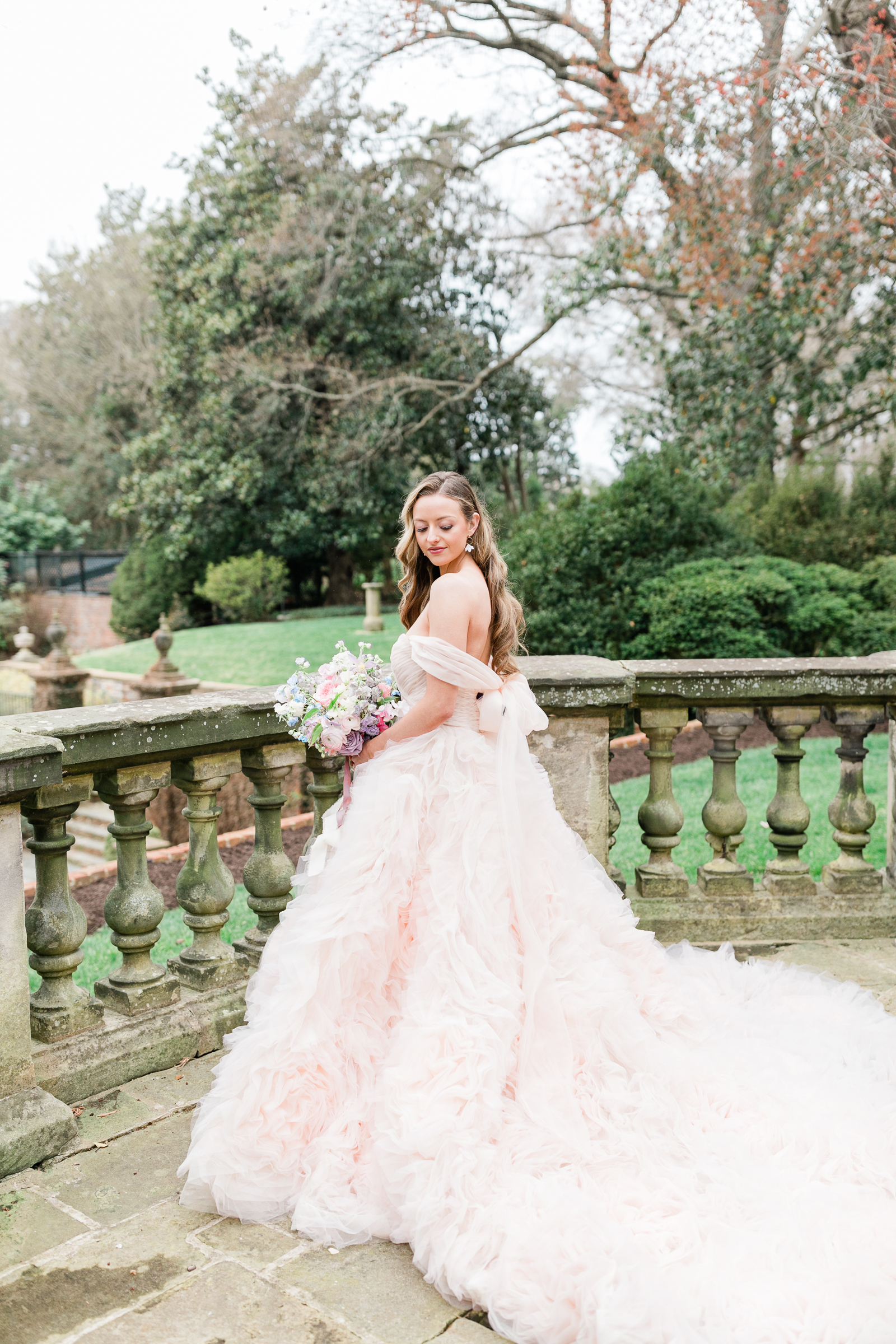The image captures a serene outdoor scene on an antique stone terrace, adorned with thick columns bearing spots of white and green mold. The terrace overlooks a lush garden filled with diverse trees, including an evergreen pine, a leafless tree, and several with pink petals, creating a picturesque backdrop. The day is sunny but with mellow, not-too-bright tones, and the sky appears washed out.

In the forefront stands a bride in a breathtaking, long, flowing wedding dress that has a light pinkish-white tint and features shoulder-less design with ample tulle. She has dirty blonde, curled long hair and dangles white earrings. The bride is looking back down at her dress, her gaze directed towards the ground with a soft, contemplative expression. In her hands, she holds a large bouquet composed of predominantly white flowers, outlined in shades of pink, adding a delicate touch to the scene. Her Caucasian complexion harmonizes with the light, peaceful atmosphere of what appears to be a beautiful day.